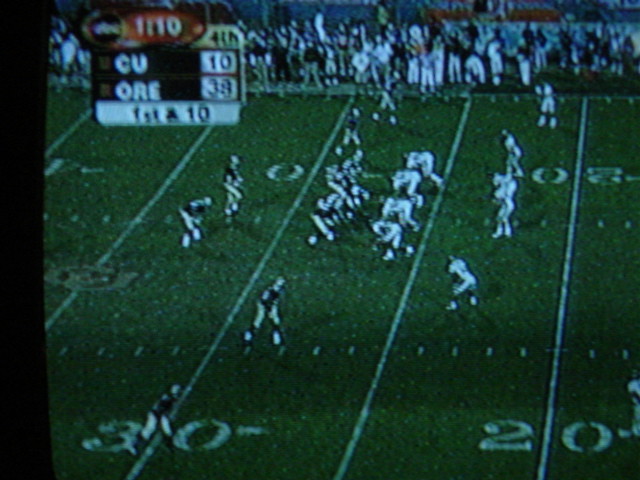The image depicts a television screen showcasing a college football game. The screen itself has an old-school design, characterized by a slightly curved black bar along the left side, which is wider at the top and bottom compared to the center.

On the field, which is visible from approximately the 30-yard line down to the 20-yard line on the closest side, the ball rests at the 27-yard line, closer to the right-hand goal. The teams are positioned as if ready to snap the ball. The team on the left side of the field is dressed in gold pants and black shirts, while the team on the right wears all-white uniforms with green letters.

In the background, a crowd of spectators fills the stands on the far side of the field. A scoreboard is displayed in the top left corner of the screen. The scoreboard has a black oval with some unreadable text, followed by a red oval which indicates the remaining game time as 1 minute and 10 seconds. The final section of the scoreboard, a yellow oval, shows that it is the fourth quarter. Below this, the score is displayed: "CU" has 10 points while "ORE" has 38 points. The information "4th and 1" is shown in a white bar with black letters underneath this score.

The entire scene captures the tension and excitement typical of a late-game moment in college football.